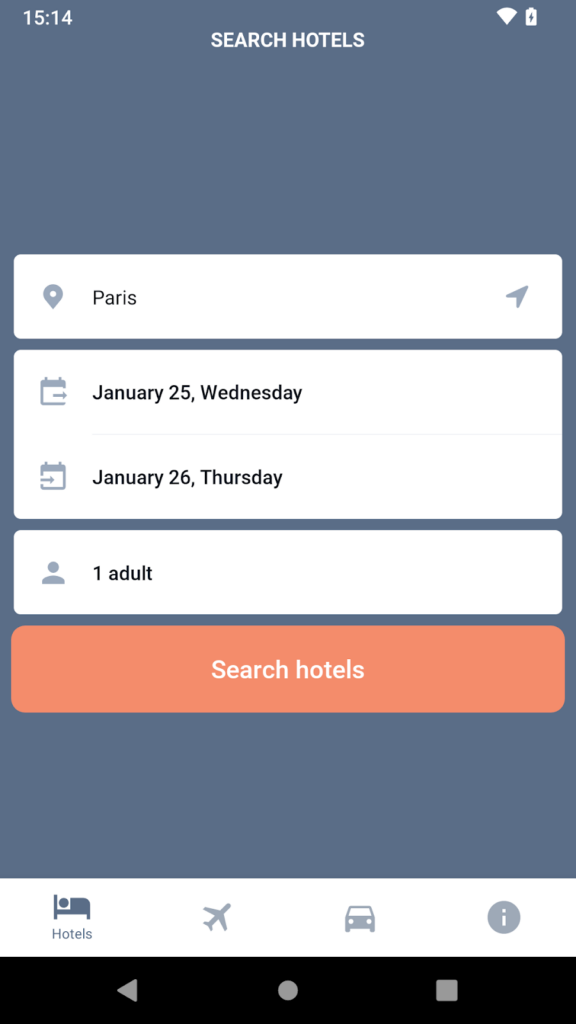The screenshot captures a phone interface taken at 3:14 AM, displaying a hotel search application. The primary background color is gray. Centered within the frame is a white text box that prominently displays the word "Paris," accompanied by a send arrow on the right-hand side. Below "Paris," the text reads "January 25th" indicating the check-in date, and "January 26th, Thursday" indicating the check-out date. The caption also notes that the search is for "one adult."

Beneath this information, there is an orange button labeled "Search Hotels." Directly underneath the gray background are various icons on a white strip, including symbols for hotels, flights, car rentals, and general information (an information circle). At the very bottom of the screen, there's a black navigation bar featuring an arrow icon for going back, a round icon for returning to the home screen, and a square icon for closing the current application.